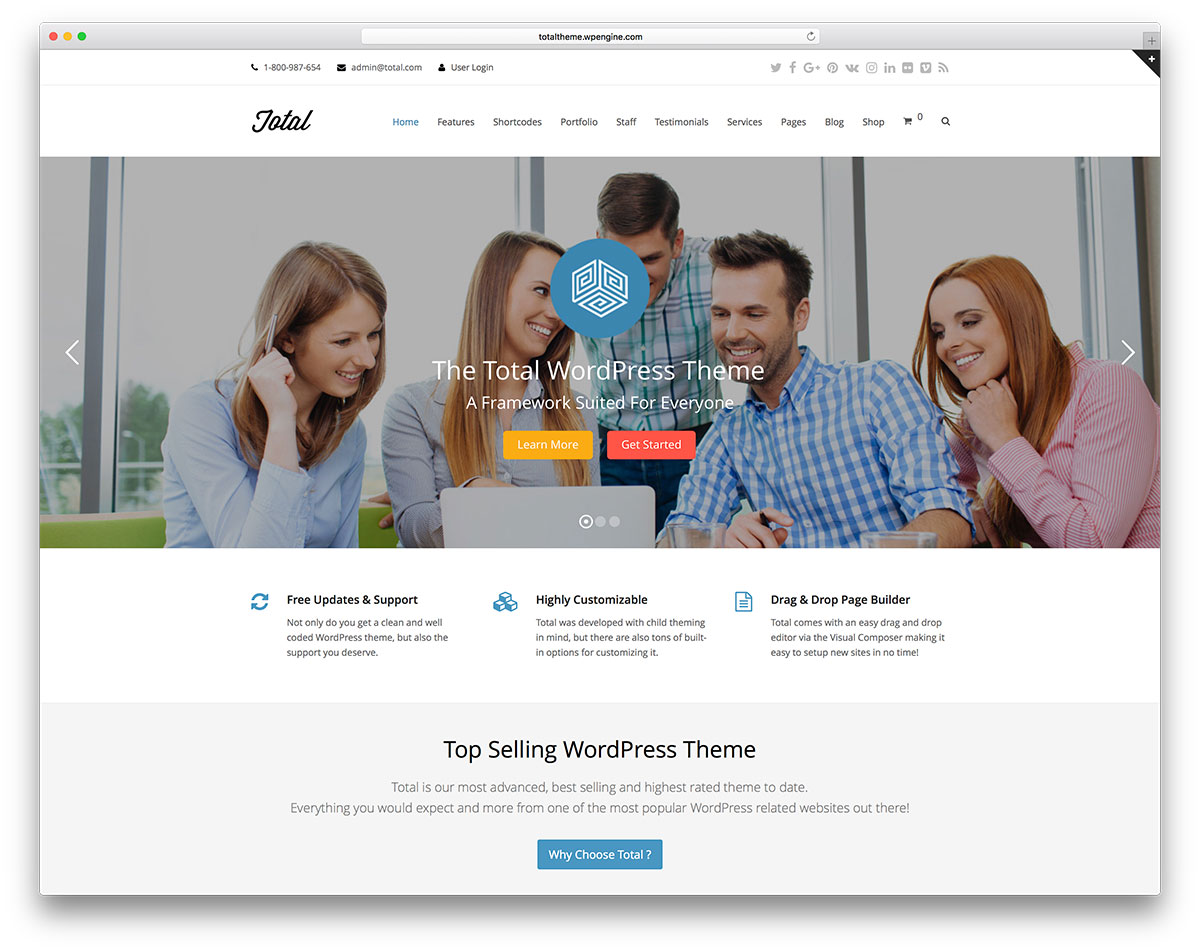The webpage presents a very inviting and professional interface. It is clearly viewed from an Apple Mac product, identifiable by the three small dots (red, orange, and green) located at the top-left corner of the browser window. The header section prominently features the website name "Total" in elegant cursive writing, alongside a search bar, and a circle with a rightward pointing arrow on the right-hand side.

Just below the header, users can find essential contact information including a phone number and email address, as well as a login option. The right side of the header includes links to the website’s social media profiles on platforms such as Twitter, Facebook, Google+, and LinkedIn.

Navigational options available in the top menu include Home, Features, Portfolio, Testimonials, Pages, and Shop. At the far end of the navigation menu, there is a shopping cart icon showing a count of zero and an additional search bar.

Dominating the central part of the webpage is an image depicting a lively scene where people are gathered around a computer, seemingly engaged in a productive discussion. The group includes two women with long dirty blonde hair on the left, both dressed in long-sleeved, buttoned-up shirts. In the center, a man stands interacting with both women and another man to the right. On the far right, a woman with strawberry blonde hair and a red striped button-up shirt attentively engages in the conversation. The overall composition of the webpage combines clear organization with appealing visual elements, providing an excellent user experience.